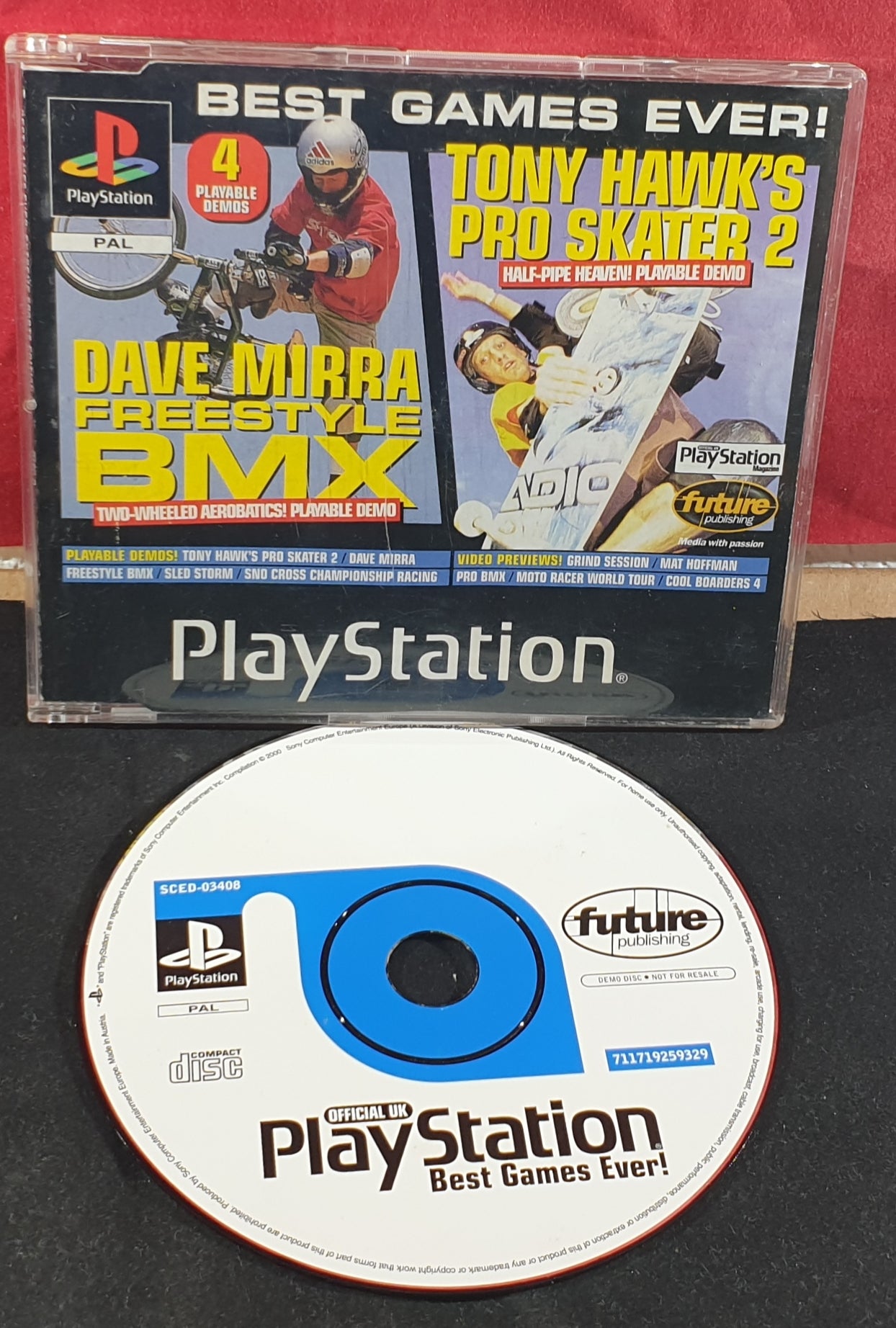This image features a classic PlayStation CD, laid flat on a black surface against a red wall. The CD itself has a white background with the text "Official UK PlayStation Best Game Ever" prominently displayed. The CD's center is a blue emblem encircling a black circle with the PlayStation symbol, and beneath this is the code SCED-03408. Adjacent to the CD is its case, which has a black background. Across the top of the case, in white text, it reads "Best Games Ever." To the right, there is an image of a skateboarder, captioned "Tony Hawk's Pro Skater 2 Half Pipe Heaven Playable Demo" in yellow text. Directly below, there's a black oval that says "Future Publishing." To the left, an image shows a person in an orange shirt with a gray helmet riding a bicycle, labeled "Dave Mirra Freestyle BMX 2-Wheeled Acrobatics Playable Demo," also in yellow text. Additional text details on the case include previews for multiple games: Grind Session, Matt Hoffman's Pro BMX, Moto Racer World Tour, and an obscured title starting with "Cool."